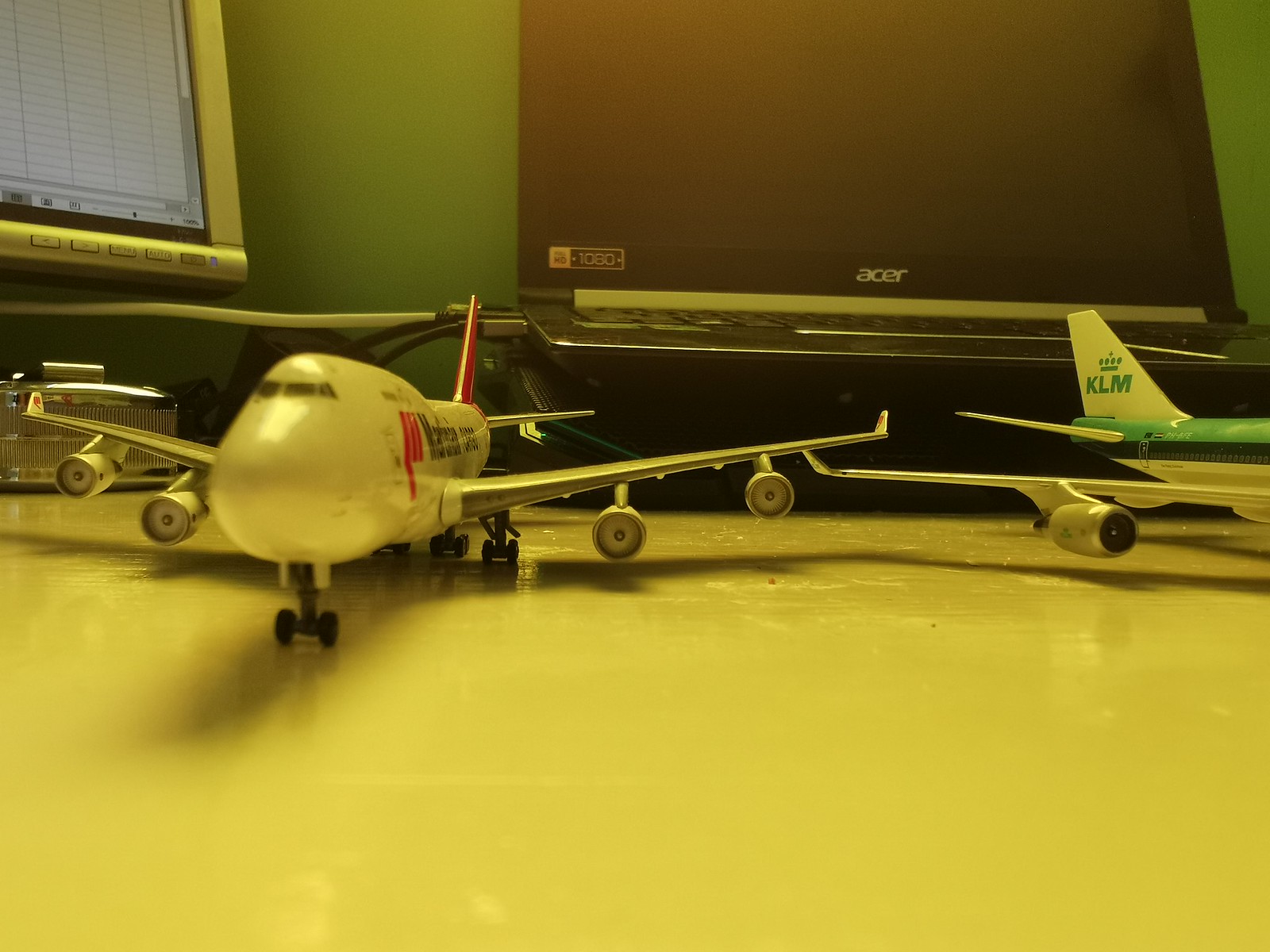The image showcases a detailed scene of a computer desk adorned with two model passenger airliners and various computing devices. The model airplane on the left is predominantly white with distinct red markings on its side and a red tail fin. The second model airplane on the right, partially visible, also features a white body with a striking black and blue stripe down the middle, branded with "KLM" and a blue crown emblem on its tail fin. The workspace includes an open Acer laptop, though it doesn't appear to be powered on, and a desktop computer located on the upper left side, displaying a spreadsheet on its screen. The lighting in the room casts a yellowish hue over the entire scene, giving it a nostalgic, warm ambiance.